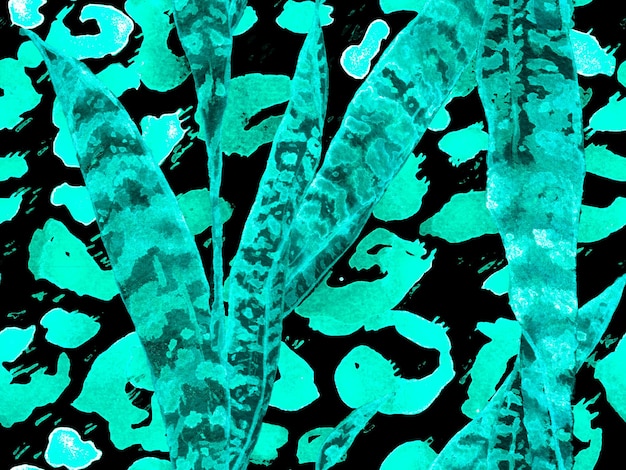This is a highly magnified, square image featuring a black background adorned with a medium green, random pattern of squiggly half-circles, potentially resembling microscopic organisms or abstract forms. Prominently, there are six elongated, narrow leaves with pointed tips superimposed over the patterned backdrop. These leaves vary in size and shade, ranging from bright green to darker green, with splotchy patterns and occasional stripes. On the left, the leaves start with a fairly large one, followed by a really skinny leaf, then a medium-sized one. At the center and toward the right, the leaves increase in size, with one large leaf and the largest one positioned on the far right alongside a shorter leaf. The arrangement of the leaves spans from the bottom left, moving upwards and slightly towards the upper right, creating a dynamic, plant-like composition over a mysterious, intricate background.